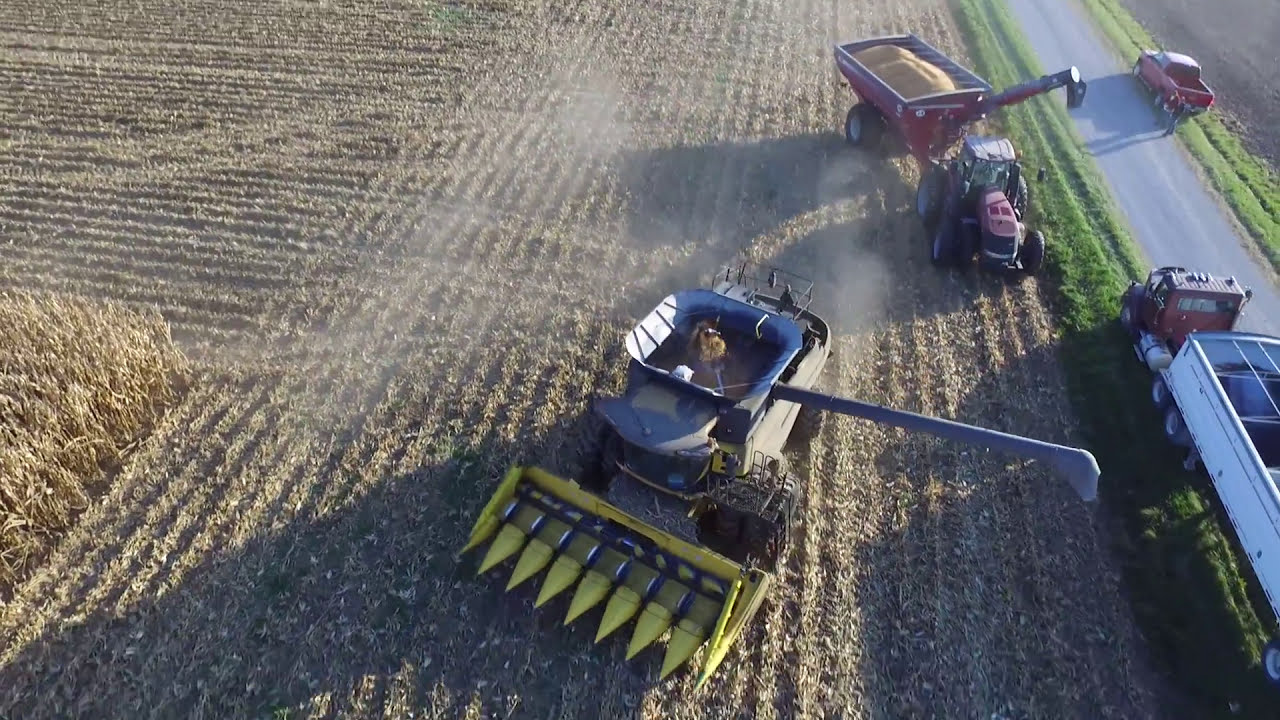The image depicts a sprawling farm field with a roadway running down its right side. On this road, a red truck is parked on a strip of grass in the upper right corner, and a larger semi-truck is located towards the bottom left of the road. The farm field on the left side of the image is actively being cultivated; a tractor is pulling a grain-filled wagon at the top of the field, while another piece of farm equipment, featuring a yellow fork and a blue arm, is actively operating in the center. The majority of the field appears to have been harvested, except for a small section on the far left edge where some crops, possibly wheat or corn, remain. The soil is visibly lined, indicating recent cultivation activity.